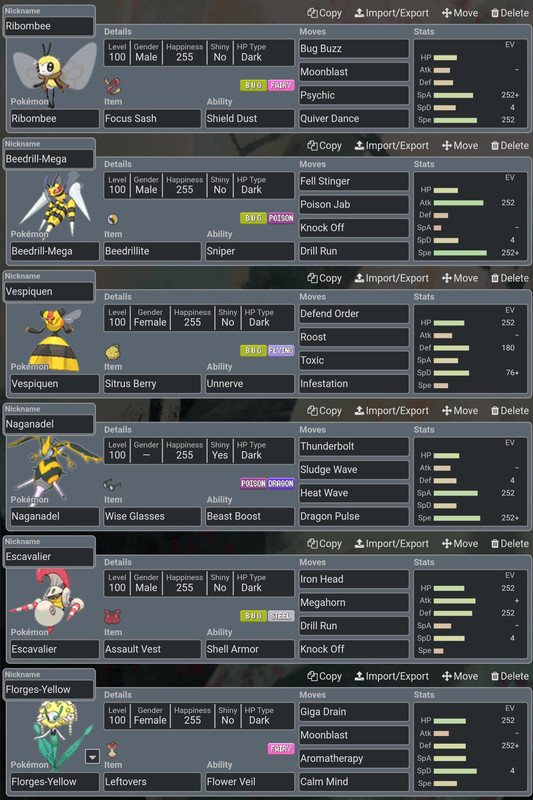This image is a detailed listing of six different Pokémon, each with specific attributes and moves. At the top of the listing are the options to Copy, Import, Export, Move, or Delete, facilitating easy management of the Pokémon data.

1. **Robibi**
   - **Level**: 100
   - **Gender**: Male
   - **Happiness**: 255
   - **Shiny**: No
   - **Type**: Dark
   - **Moves**: Bug Buzz, Moon Blast, Psychic, Quiver Dance
   - **Stats**: Detailed specifics not shown in the description

2. **Buildery Mega**
   - **Level**: 100
   - **Gender**: Male
   - **Happiness**: 255
   - **Shiny**: No
   - **Type**: Dark
   - **Item**: Buildery Light
   - **Ability**: Sniper
   - **Moves**: Fell Stinger, Poison Jab, Knock Off, Drill Run
   - **Stats**: Detailed specifics not shown in the description

3. **Vespi Queen**
   - **Level**: 100
   - **Gender**: Female
   - **Happiness**: 255
   - **Shiny**: No
   - **Type**: Dark
   - **Moves**: Defend Order, Roost, Toxic, Infestation
   - **Stats**: Detailed specifics not shown in the description

4. **Nagadel**
   - **Level**: 100
   - **Gender**: Genderless
   - **Happiness**: 255
   - **Shiny**: No
   - **Type**: Dark
   - **Moves**: Details not provided
   - **Stats**: Detailed specifics not shown in the description

5. **Escavalor**
   - **Level**: 100
   - **Gender**: Male (assumed from context)
   - **Happiness**: 255
   - **Shiny**: No
   - **Type**: Dark
   - **Moves**: Details not provided
   - **Stats**: Detailed specifics not shown in the description

6. **Flourish Yellow**
   - **Level**: 100
   - **Gender**: Female (assumed from description)
   - **Happiness**: 255
   - **Shiny**: No
   - **Type**: Dark
   - **Moves**: Details not provided
   - **Stats**: Detailed specifics not shown in the description

The Pokémon listed exhibit a thematic connection to bees and related structures, with names and characteristics suggestive of bees, hive queens, and floral elements. This cohesive theme adds an interesting layer to the collection, making it aesthetically and narratively appealing.